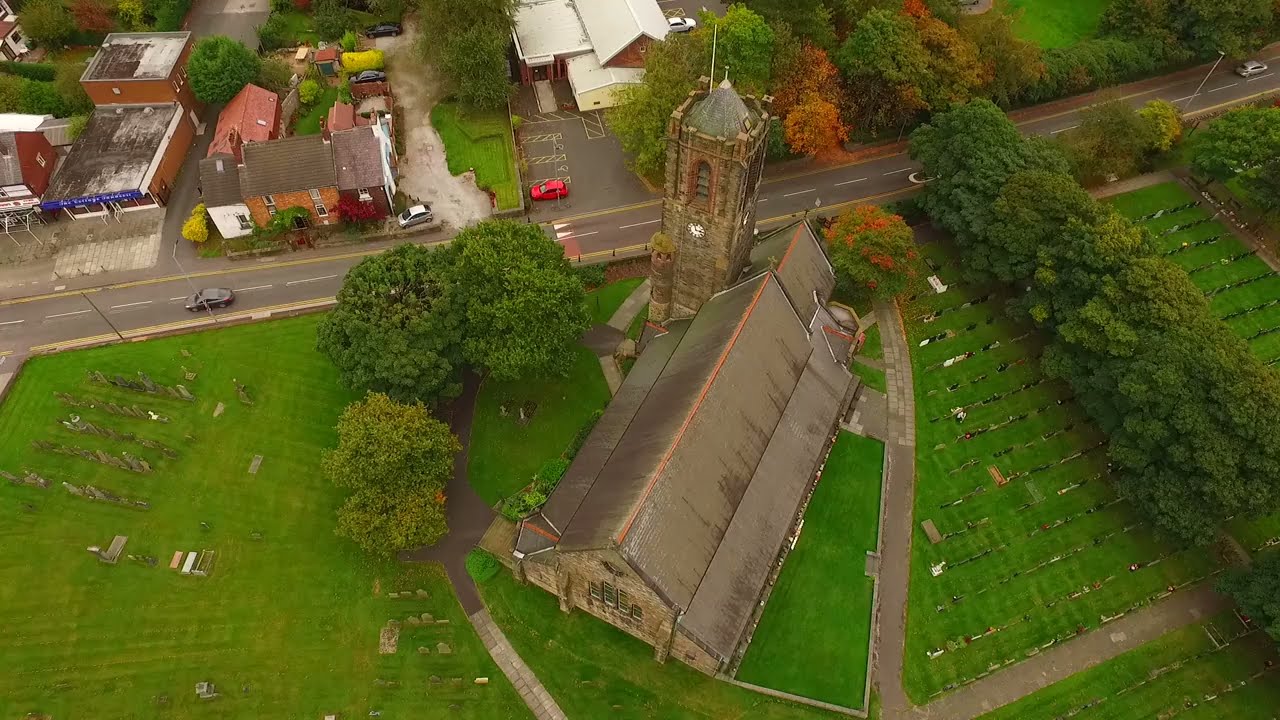This aerial shot captures a picturesque, likely East Coast setting centered around an old stone church, showcasing its age and detailed architecture. The church's roof, divided into two peaked sections with a bisecting line, is likely designed for snow shedding. The roof, gray in color, converges into a tall tower that might be a clock tower, featuring domed windows that could be stained glass, and topped with a cross. Surrounding the church, a gray stone walkway encircles the structure, leading out to a paved roundabout that connects to a main road stretching from the upper left to the lower right of the image. 

Behind the church, there is a distinctive tall silo-like structure, reinforcing the historic and possibly agricultural vibe of the area, though it might alternatively suggest a tower commonly found in church designs. To the lower right, a dense row of green trees marks the boundary of a cemetery, with horizontal rows of tombstones suggesting a serene resting place. The cemetery appears to extend to the left side, merging into a large green field dotted with more tombstones and some parking lots. Scattered nearby buildings blend into the rustic charm, adding to the overall farm-like ambiance. 

Notably, the scene includes a mix of autumn foliage, hinting at the seasonal shift, and a variety of parked cars, including white, darker-colored, and a red vehicle, situated in a lot to the left of the church. Together, these elements paint a comprehensive picture of a historical church surrounded by natural beauty, a serene cemetery, and hints of a rural community.